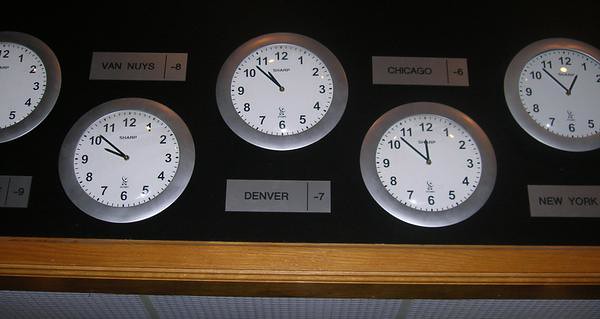This image captures a wall adorned with a series of five clocks against a chocolate brown backdrop, each clock accompanied by a silver horizontal band indicating various city names. The photograph is taken from a slightly lower angle, giving the impression that the wall is gently tilting backward. At the very bottom of the image, a thin strip of white wall is visible, just above which lies a horizontal line of maple-colored wood trim.

Starting from the left, the upper left clock is partially cut off, obscuring both the time and the city label. Directly below it, in the down position, is a clock labeled "Van Nuys," showing the time as 9:50. Moving to the center, the clock positioned higher up is labeled "Denver" with the current time of 10:53. Below and to the right of the Denver clock, the "Chicago" clock shows 11:53. Finally, at the upper right corner, the clock labeled "New York" indicates the time as 12:53. The arrangement of the clocks, staggered alternately up and down with their respective city labels, creates a dynamic and intriguing visual layout on the wall.